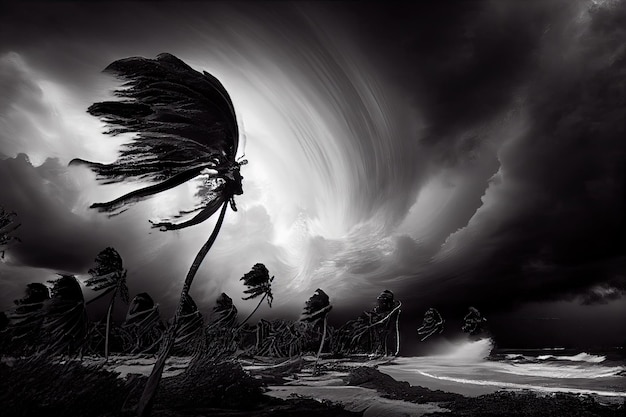This highly detailed black and white illustration depicts a turbulent storm on a beach lined with numerous palm trees. The scene's central focus is a large palm tree in the foreground, with its slender trunk and abundant fronds blown sharply to the left by the fierce wind. Surrounding it are eleven shorter palm trees, all similarly wind-swept, their profiles evoking the sensation of intense gusts. The background showcases a swirling sky, marked by dark, ominous clouds interspersed with areas of light that enhance the dramatic feel. This vortex of clouds forms a distinctive U-shape, with darker, more solid clouds to the left and lighter, more ethereal spirals towards the center. The right side of the image features a stormy ocean, its choppy waves crashing violently against the shore. Some waves obscure the bases of the closest palm trees, adding to the chaotic environment. The shoreline also displays a mix of foliage, possible seaweed, and rocky formations. Overall, the blending of dark and light tones, coupled with the dynamic motion of the elements, underlines the illustration's intense and almost palpable depiction of a storm’s fury.